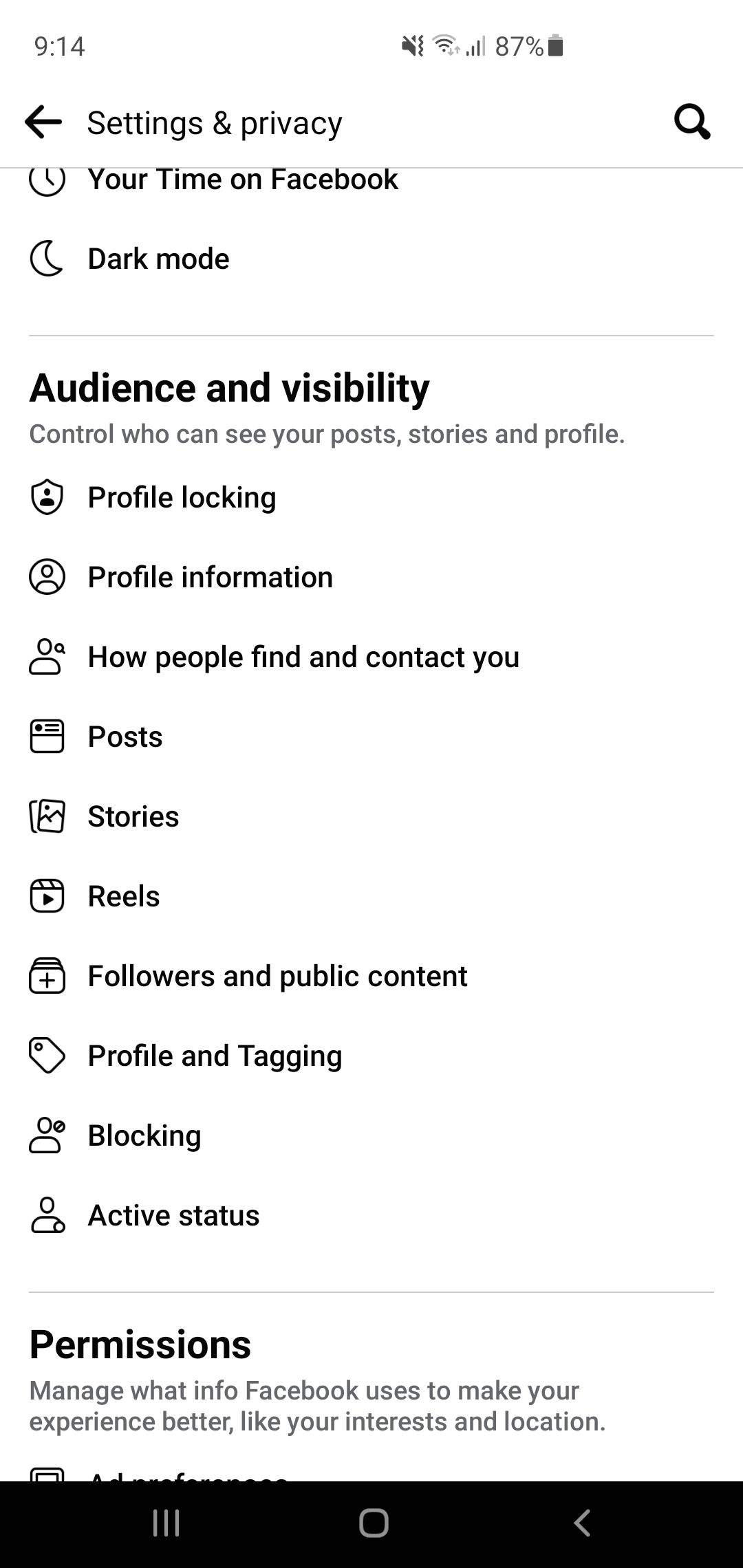In this screenshot taken from a smartphone, the top section of the image displays the phone's status bar, which shows the battery life at 91% and other typical icons. Directly beneath the status bar, there is a "Settings & Privacy" section with an option to navigate back. The page heading is "Your Time on Facebook," accompanied by a clock icon, and next to it is a "Dark Mode" option symbolized by a moon.

To the right of the "Settings & Privacy" title is a magnifying glass icon, indicating a search functionality. A horizontal line separates this header from the main content below.

The subsequent section addresses privacy controls, starting with "Control who can see your posts, stories, and profile." It includes a "Profile Locking" option represented by a badge icon. Other options in this section include "Profile Information," managing how people find and contact you, and settings for "Posts, Stories, Reels, Followers, and Public Content." Each option is accompanied by a relevant emoji to enhance understanding visually.

Following these options, another horizontal separator line leads to the "Permissions" section, which allows users to manage the information Facebook uses to tailor their experience, such as interests and location data.

At the very bottom of the page, there are three icons: three vertical lines on the left, a square in the middle, and a back button on the right. These likely serve as navigation controls within the app.

The detailed arrangement and icons aim to enhance user navigation and control over their Facebook privacy and experience settings.